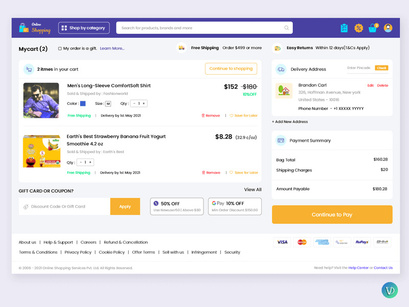A dark-themed shopping website is displayed, predominantly featuring colors of dark blue, orange, and white. At the top of the page, a dark blue border includes a partially illegible word in white text, with the visible word "shopping" rendered in bright orange. The website design incorporates various icons in either blue or orange, maintaining the color scheme throughout.

The user interface includes a "Shop by Category" option and a bright white search bar for easy navigation. A cart icon indicates that there are currently two items inside. Users have the option to mark items as gifts and are informed about free shipping for orders totaling $499 or more. The customer's name, though difficult to read, appears at the top along with the delivery address.

Detailed content of the cart reveals two items: 
1. A man's long-sleeve comfort shirt in blue, size medium, priced at $152.
2. "Earth's Strawberry Banana Fruit Yogurt Smoothie," featuring Elmo on the packaging, priced at $8.28 each.

The website offers several promotional deals:
- 50% off when paying with an unspecified method
- 30% off when using Google Pay.

Additional options include applying a gift card or coupon. Below these offers, the layout shows shipping charges, the total purchase amount, and the button to proceed to payment. Accepted payment methods are widely inclusive, accepting Visa, MasterCard, American Express, and several others.